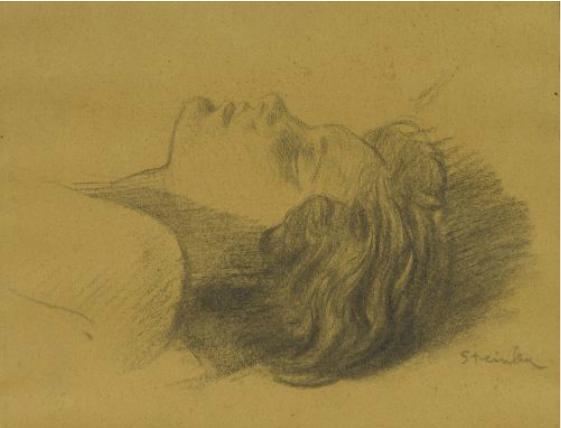This detailed pencil sketch, rendered on dark yellow or manila paper, portrays a serene woman lying back with her eyes closed, suggesting sleep or deep rest. Her head is tilted upwards, facing the sky, with a gentle, peaceful expression. She has short to medium-length, fluffy hair that cascades back, casting a shadow beneath it due to an off-screen light source. Her face is seen in profile, revealing a strong chin, a small pointy nose, and balanced lips. Only one of her shoulders is visible, blending into the unfinished sketch that fades into the void. The piece also showcases a bare shoulder and a glimpse of her arm. Subtle pencil shading creates depth and shadow, enhancing the tranquil atmosphere. At the bottom right of the drawing, there is a partially legible signature, possibly reading "STINLER" or something similar.